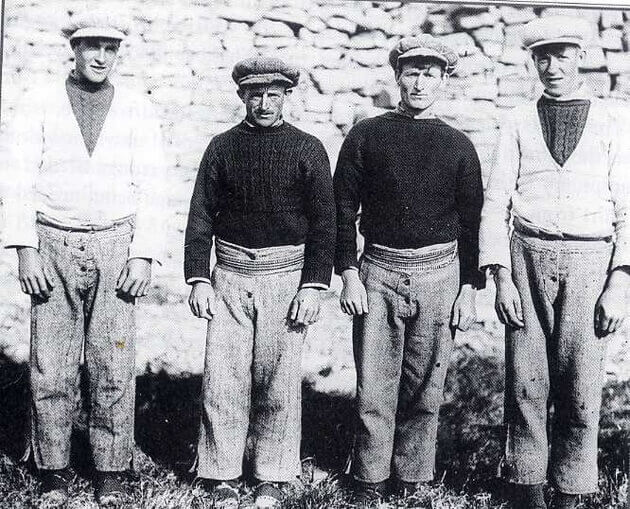This is a detailed black and white photograph from the early 1900s, capturing four Caucasian men standing side by side on a grassy field in front of a tall stone wall. The scene, reminiscent of early 20th century Britain or Ireland, features the men, who are of varying heights, dressed in what appears to be traditional labor or farm attire of that era. All four are donned in loose-fitting wool trousers and layered, thick long-sleeve knit sweaters. Specifically, the men on the left and right edges of the photograph wear white v-neck sweaters over dark, cable-knit sweaters, while the two men in the center sport dark knit sweaters. Each man also has a large billed cap, characterized by a wide, somewhat puffy design with the visor rising just above their eyes. Although they resemble individuals you might find at a horse racing event, perhaps jockeys or farm workers, they are all wearing standard work shoes rather than boots. The photograph, devoid of any text, encapsulates a snapshot of attire and outdoor life from over a century ago.